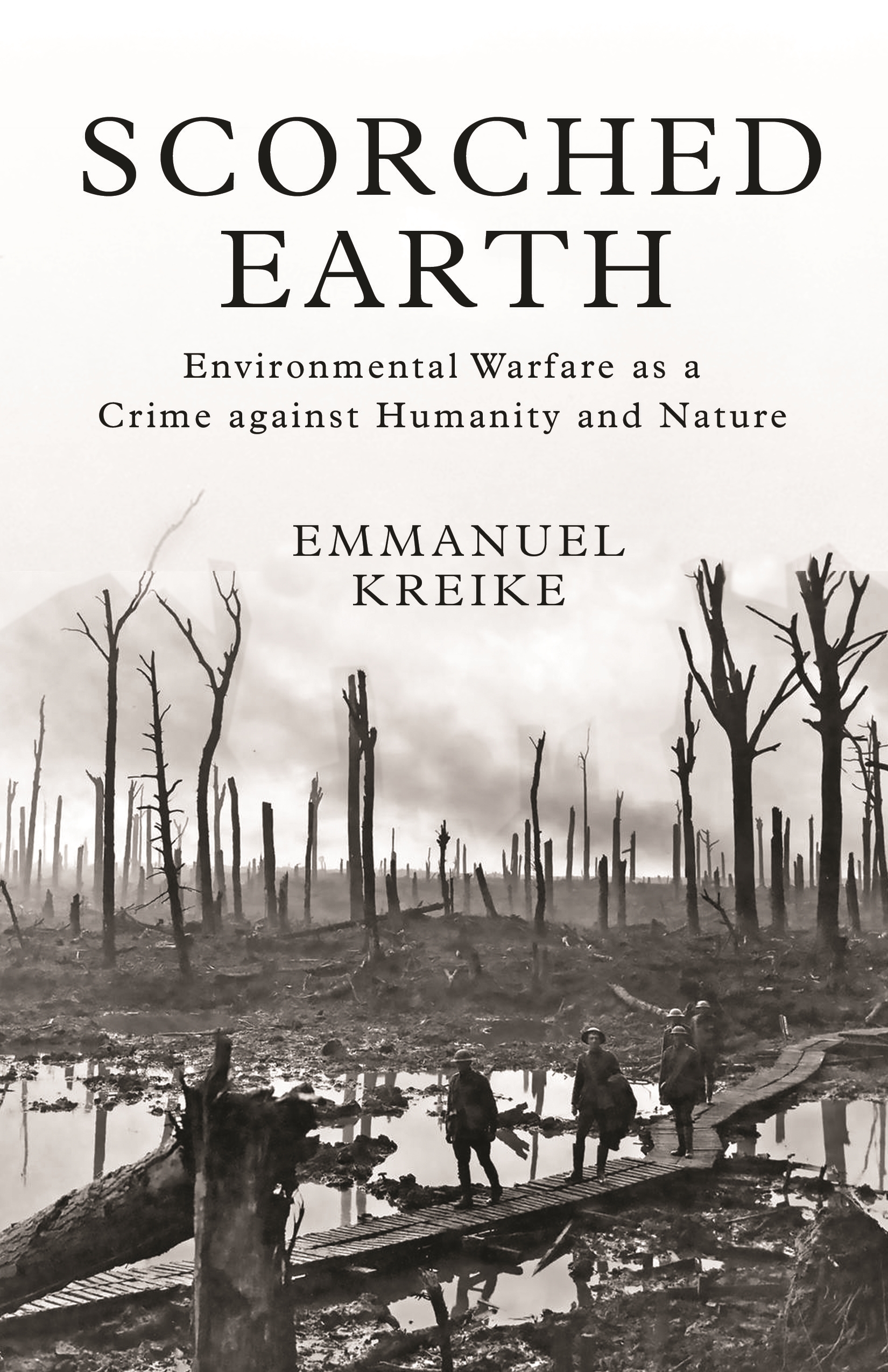The image appears to be the cover of a book titled "Scorched Earth: Environmental Warfare as a Crime Against Humanity and Nature" by Emanuel Krake. Set against a predominantly black and white or gray and white background, the stark imagery below the title depicts a desolate, burned-out forest. Leafless, scorched trees with truncated branches tower around what used to be a verdant landscape, now reduced to a wasteland with a very cloudy, smoky sky overhead. In the foreground, a small, low wooden bridge extends across a body of water, possibly a pond or lake, creating a makeshift pathway through the devastation. Three figures, appearing as men, stand on the bridge, gazing into the distance, embodying the somber tone of deforestation and environmental wreckage.